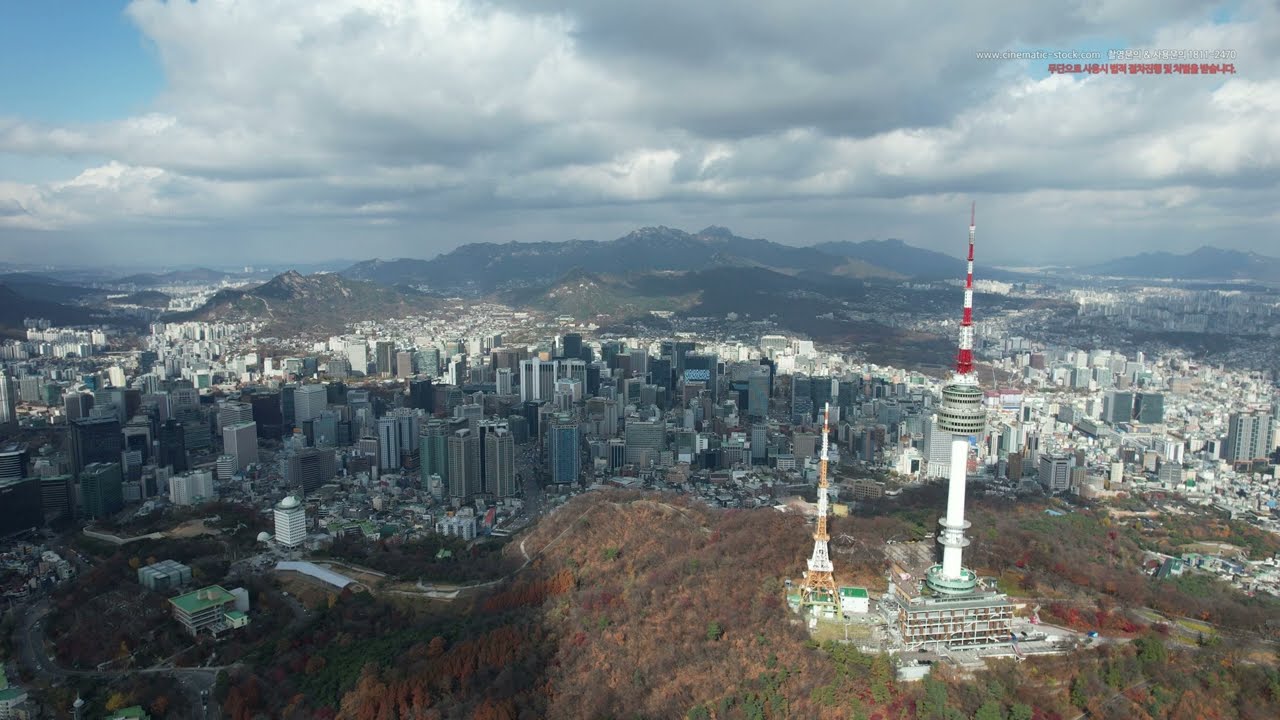This aerial photograph captures a bustling city nestled in a mountainous region, possibly somewhere in East Asia, given the architectural style and Korean text watermark that reads "www.cinematic-stock.com". The image has a dramatic, almost postcard-like feel, dominated by a moody sky with heavy, gray clouds casting shadows over the urban landscape.

In the foreground, the cityscape is punctuated by two distinctive tower structures. The one on the right resembles Seattle's Space Needle and features an observation deck adorned with red and white stripes at the top, perched on a platform. To its left stands a smaller tower, reminiscent of a mini Eiffel Tower. Both structures may serve as radio towers and are surrounded by hills dotted with red and orange foliage, suggesting a fall setting.

The city itself is densely populated with a plethora of tall, grey, metallic-looking apartment buildings, although not quite reaching the heights of traditional skyscrapers. The buildings diminish in height toward the edges of the photo, giving way to more residential and possibly tourist-friendly natural areas. The mountainous backdrop and the dramatic sky further accentuate the city's scenic and somewhat somber atmosphere.